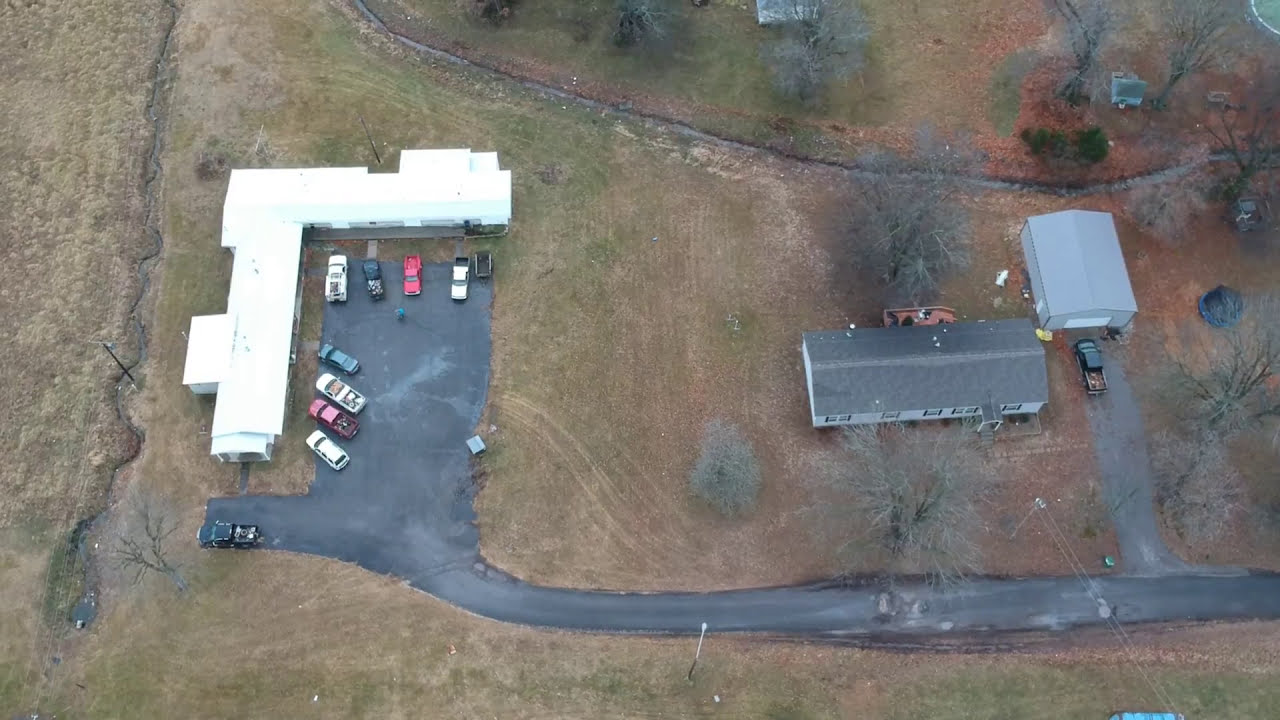This aerial photograph captures a rural property from a significant height, likely taken with a drone. The focal point of the image is a single road that runs horizontally along the bottom edge, transitioning into an asphalt driveway which extends vertically and curves towards a building cluster. In the center right of the image, there is a light blue, one-story house with dark gray shingles. Adjacent to this house is a small, rectangular gray building with a white garage door, in front of which a dark green truck is parked, possibly with wood in its bed.

Further left, the driveway expands into a larger rectangular parking area around an L-shaped, white-roofed building. This upside-down L-shaped structure is the largest on the property and is surrounded by eight to ten vehicles. The surrounding area features a mixture of dirt and patchy grass, giving the land an off-green hue. Sparse, leafless trees dot the landscape, suggesting the photograph was taken during winter.